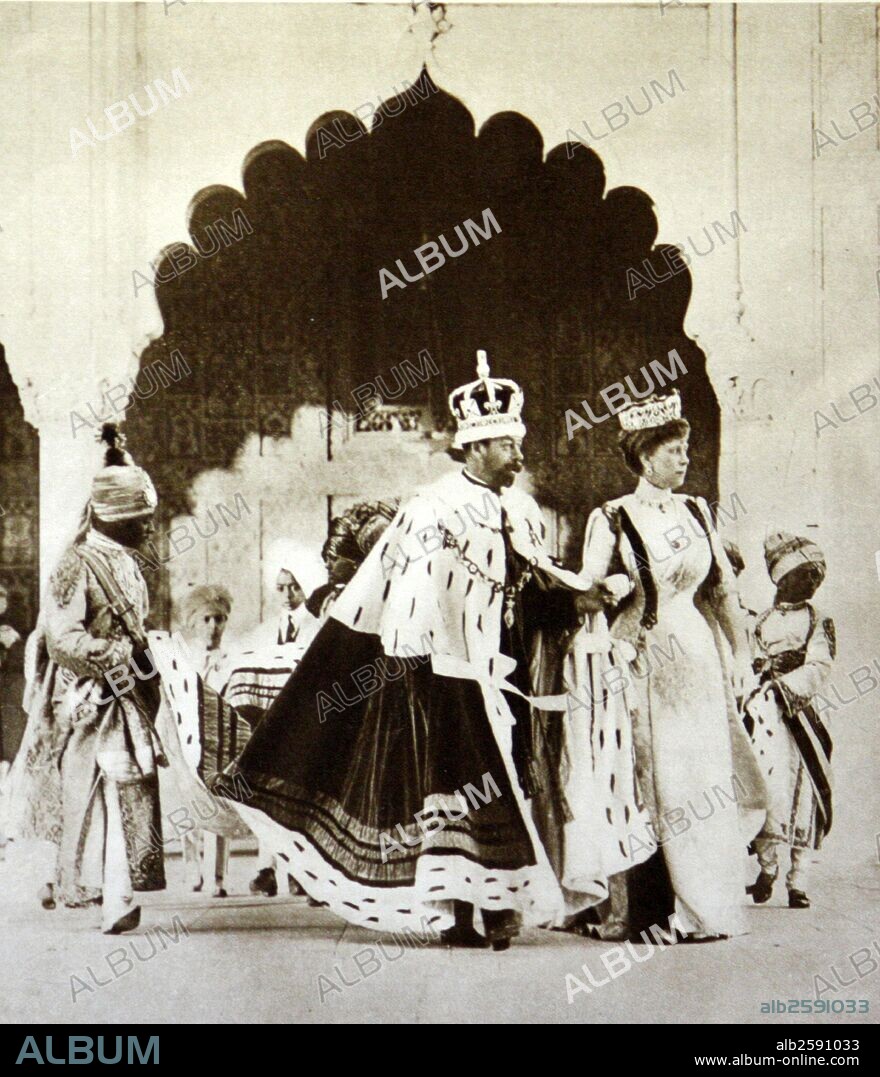This detailed black-and-white photo depicts what appears to be King George of England and the Queen, both adorned with ornate crowns and regal attire. The King is distinguished by his ornate British-style crown and a luxurious robe with a white cape featuring vertical black lines, transitioning to a black skirt. He holds the Queen's hand, who wears a narrower crown and a long white dress. The background suggests a setting in India, as there are several figures dressed in traditional Indian or Hindu clothing, including a man in a large turban. The couple stands upright, possibly under a decorated arch, with the surrounding figures not directly facing the camera. The entire image is stamped repeatedly with the word "album."